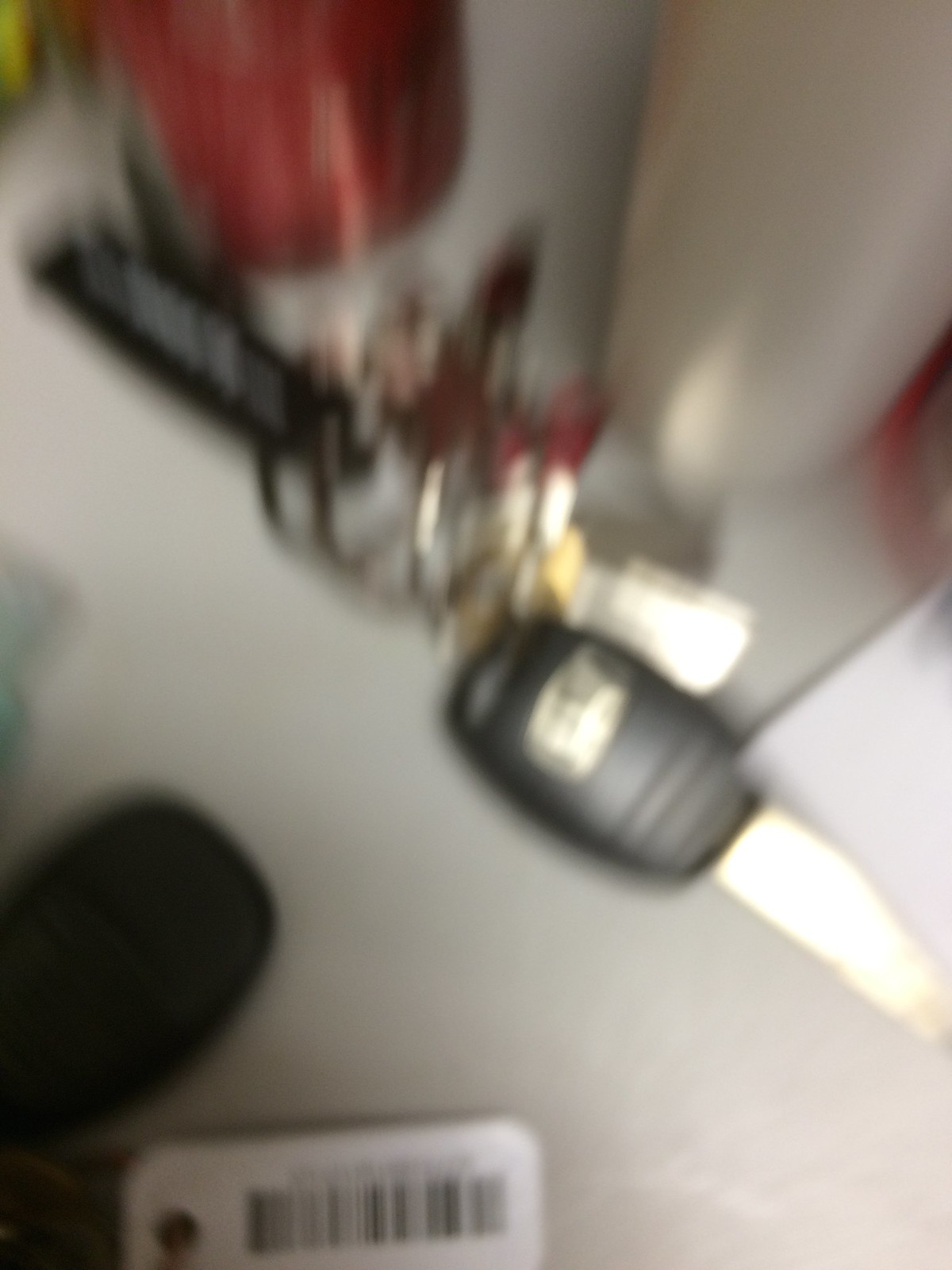This photograph, although slightly blurry, captures various items arranged on a white tabletop or countertop. On the left side of the table, there is a set of keys featuring a black key fob, likely for a car, attached to a keyring that includes a white, rectangular piece of plastic. This plastic piece appears to have a UPC code, suggesting it could be a rewards card for a grocery store. While the lettering on the UPC code is unreadable, its presence is distinct. Adjacent to this, another set of keys is present, also with a black key fob and a gold-colored key that has a similarly hued sticker on it, though its details are indistinguishable. Additionally, there seems to be a metal object with a corkscrew-like design resting on the table. Completing the scene, a red can, possibly soda, sits on the tabletop adding a touch of color to the otherwise monochromatic setting.